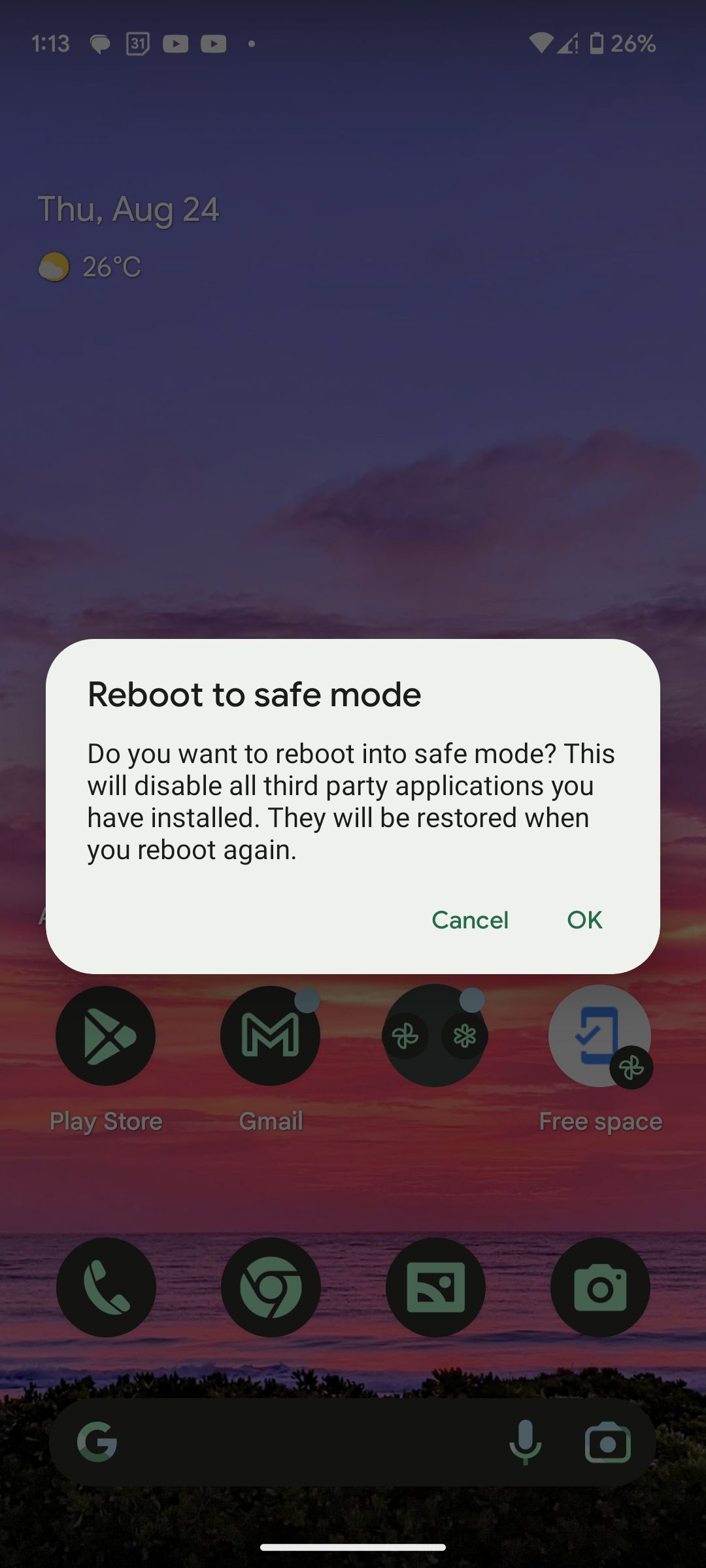This smartphone screenshot captures a serene dusk screensaver, depicting a picturesque scene of tree silhouettes and a waterway under a vividly colored twilight sky. The upper portion of the screen displays a digital clock showing 1:13, accompanied by two conversation bubbles, a circular icon with the number 31, and two YouTube logos. To the right, symbols for Wi-Fi connectivity and a battery indicator showing 26% charge are visible.

Below the time, on the left side, the date, "Thursday, August 24th," is prominently displayed alongside a partly sunny weather icon indicating a temperature of 26 degrees Celsius. A white pop-up box overlays the main display, posing the question, "Reboot to safe mode? Do you want to reboot into safe mode? This will disable all third-party applications you have installed. They will be restored when you reboot again." There are two action buttons, "Cancel" and "OK."

The home screen beneath the pop-up features various app icons, including the Play Store, Gmail, a mysterious fan-like icon with an atomic symbol, a telephone, Google, Photos, and a camera. Another Gmail icon is also present, along with a search box that includes a microphone and camera symbol, hinting at the multifunctional capabilities of the device's search features.